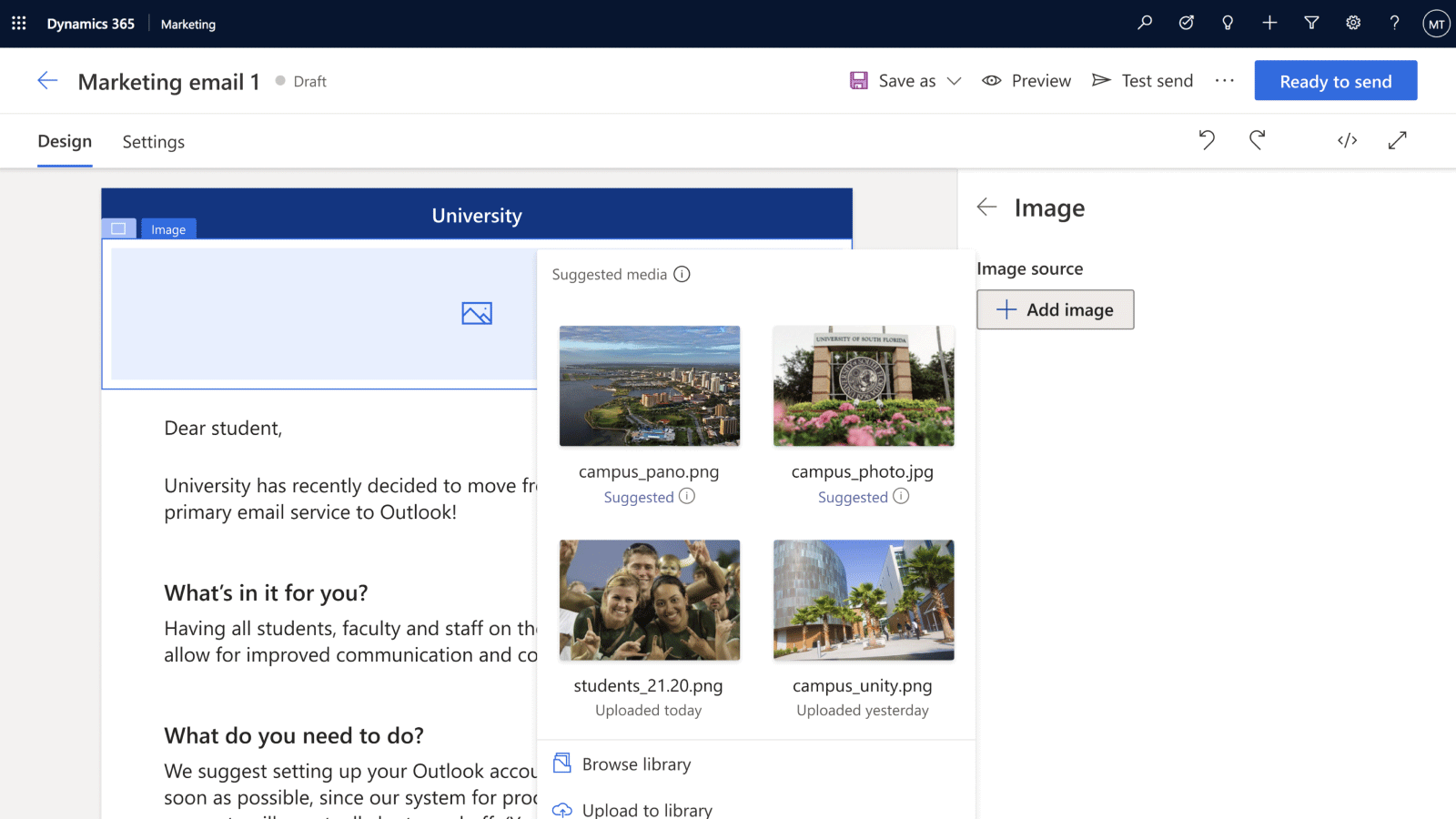This image depicts a web page from the "Dynamic 365 Marketing" platform. The top toolbar of the website features a dark navy blue banner with "Dynamic 365 / Marketing" prominently displayed in the upper left corner. On the right side of this toolbar, multiple icons can be seen: a search icon, a gear icon for settings, a question mark icon for help, and a white circle displaying the initials "MT," likely indicating the logged-in user's username.

Below the toolbar, the upper section of the page displays the title "Marketing Email 1" followed by the label "Draft," indicating that this email is currently in draft form. To the right of this title, there are buttons for "Save As," "Preview," and "Test Send." Additionally, a blue "Ready to Send" button is located further to the right.

The main content area of the page is set to the "Design" tab, which is currently active. Adjacent to the design tab is the "Settings" tab, which is not selected. The design tab layout begins with the placeholder text "university" at the top and a blank image field, ready for an image to be inserted. The email template within the design area includes sections titled "Dear Student," "What's in it for you?" and "What do you need to do?" suggesting a format for drafting mass marketing emails.

Additionally, the page offers a selection of suggested media files, listed as "campuspiano.png," "campusphoto.jpg," "students.png," and "campusunity.png," which can be used to enhance the email design.